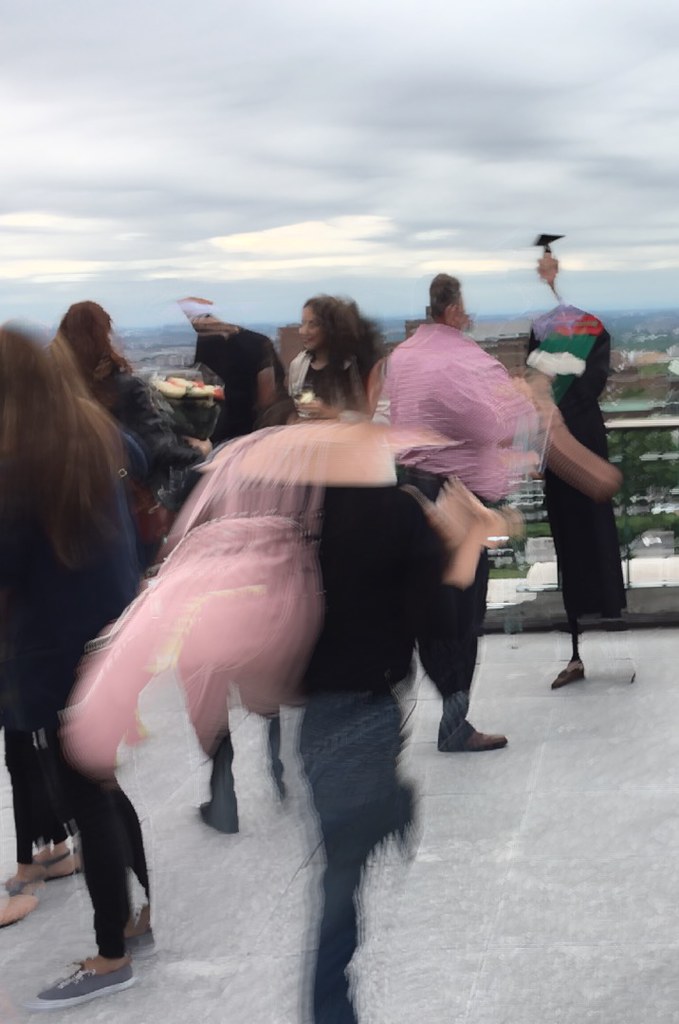This AI-generated image depicts a group of seven indistinguishable individuals standing on a patio with a railing, overlooking a cloudy cityscape. One person appears to be wearing a graduation gown, while the others are blurred and lack distinct features such as faces, hands, and feet. The scene is highly distorted, with people and objects blending into one another, making it difficult to discern any specific details. The overall composition of the photo is abstract and surreal, characterized by missing limbs and a general sense of morphing.